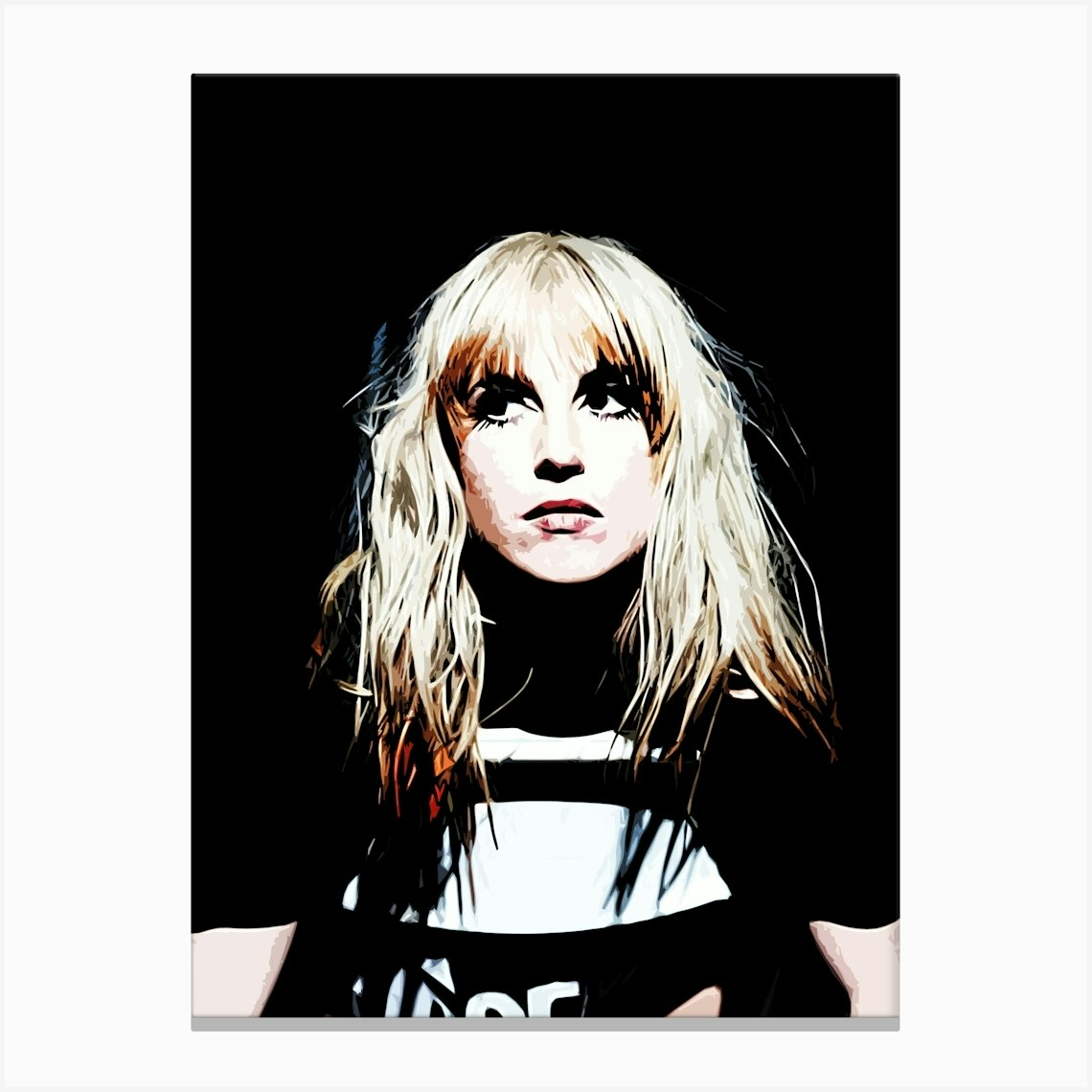The image is a vector illustration resembling a cell-shaded portrait of Hayley Williams from Paramore. The artwork features distinct layers to achieve depth and color differentiation. Hayley, a Caucasian woman with long blonde hair featuring copper tips, is centrally positioned and facing the viewer, though her gaze is directed slightly to the left. Her hair cascades just below her shoulders. The background is pitch black, making her black and white shirt blend seamlessly into the darkness, creating an illusion where only her hair, face, and a bit of her shirt are clearly visible. The entire composition is framed by a light gray background with a darker gray border. Her face is illuminated brightly, suggesting a spotlight effect in a dark room. She is wearing eye makeup and lipstick that highlights her features, while subtle blue shades appear in her hair, adding to a grunge, artistic vibe. Across the bottom of her outfit, there are some white letters, adding a small detail to her ensemble. The overall format of the image is almost square with a notable black rectangle in the center, framed by lighter tones on the edges.